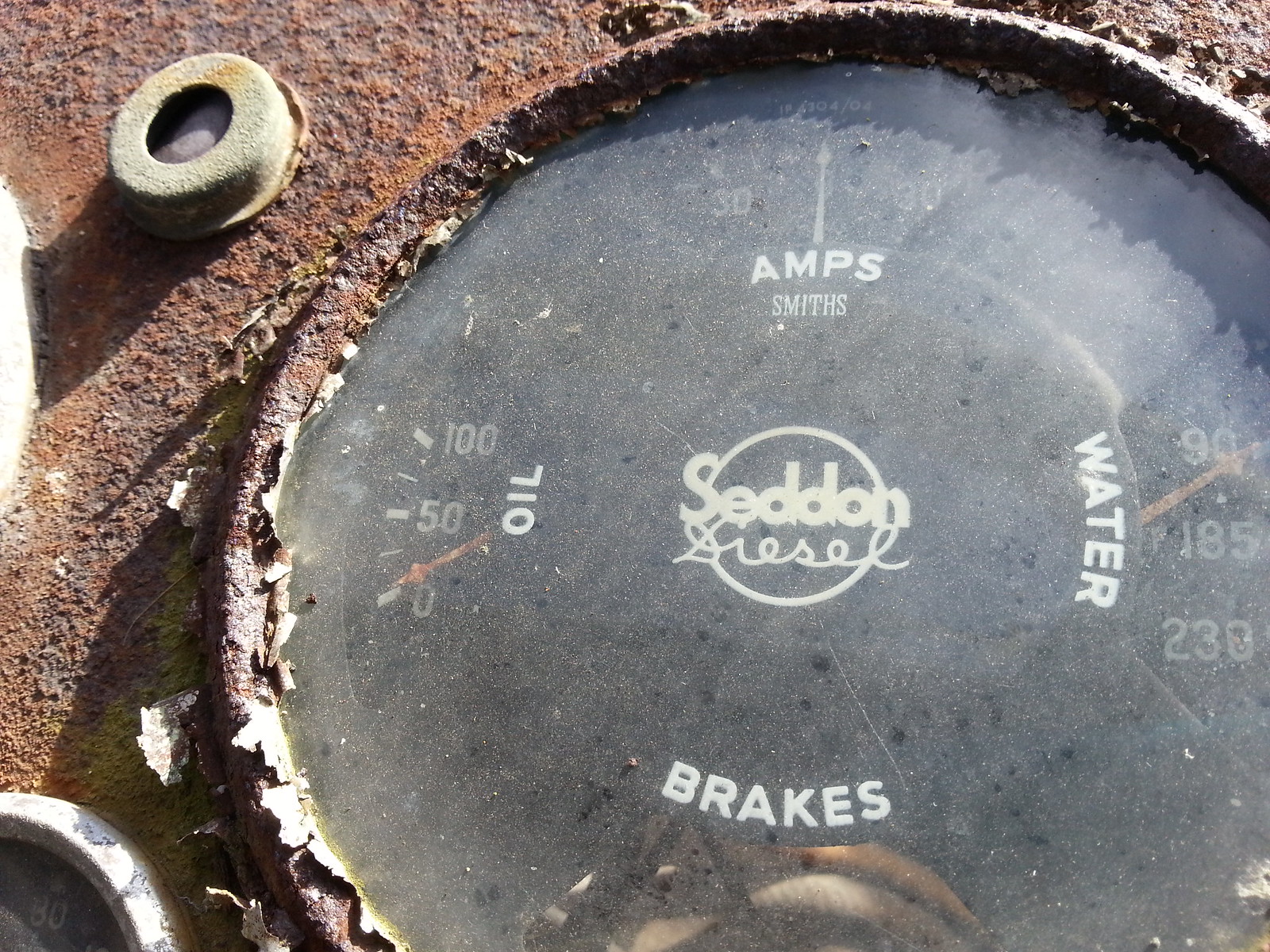This photograph features a vintage gauge panel from a Seddon diesel equipment. The rusted, worn-out panel houses an array of meters, each telling a story of a time long past. The primary gauge displays an ammeter and a water level indicator, with levels marked at 90, 185, and 230. A partially obscured brake indicator rests at the bottom of the gauge, its meaning shrouded by the curled nature of the label. Another critical instrument is the oil pressure gauge, which ranges from 0 to 100 with intermediate markings at 25, 50, and 75. Notably, both the ammeter and the oil pressure gauge show no readings, hinting that the equipment is currently off. The glass covering the gauges is cloudy but remains intact, adding to the nostalgic charm of this antiquated piece.